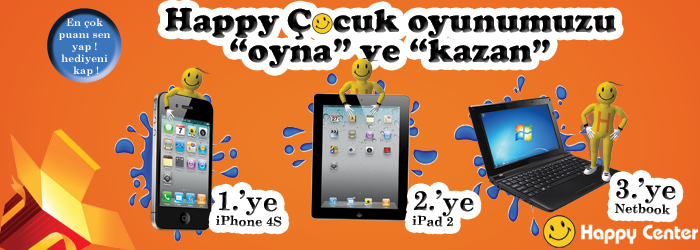The advertisement features a vibrant medium-orange background with an open red box in the bottom left corner, its yellow lids revealing a bright white reflection at the center, resembling a shining gift. Toward the top of the page, the text "Happy" is followed by a playful replacement of the letter "O" with a tilted yellow smiley face, creating the word "Cocuk Oyunumuz" in an unfamiliar language. Below, in quotes, it reads "Oyna ve Kazan" meaning "Play and Win." On the right, the ad showcases three electronic devices: an iPhone 4S on the far left with cartoonish water splashes and a smiley face character, an iPad 2 in the middle with similar graphics, and a netbook laptop with a Windows background on the right, labeled with sequential numbers "1.'ye," "2.'ye," and "3.'ye," respectively. The bottom right corner displays additional text with another tilted smiley face and the phrase "Happy Center," suggesting the promotional context for these devices.